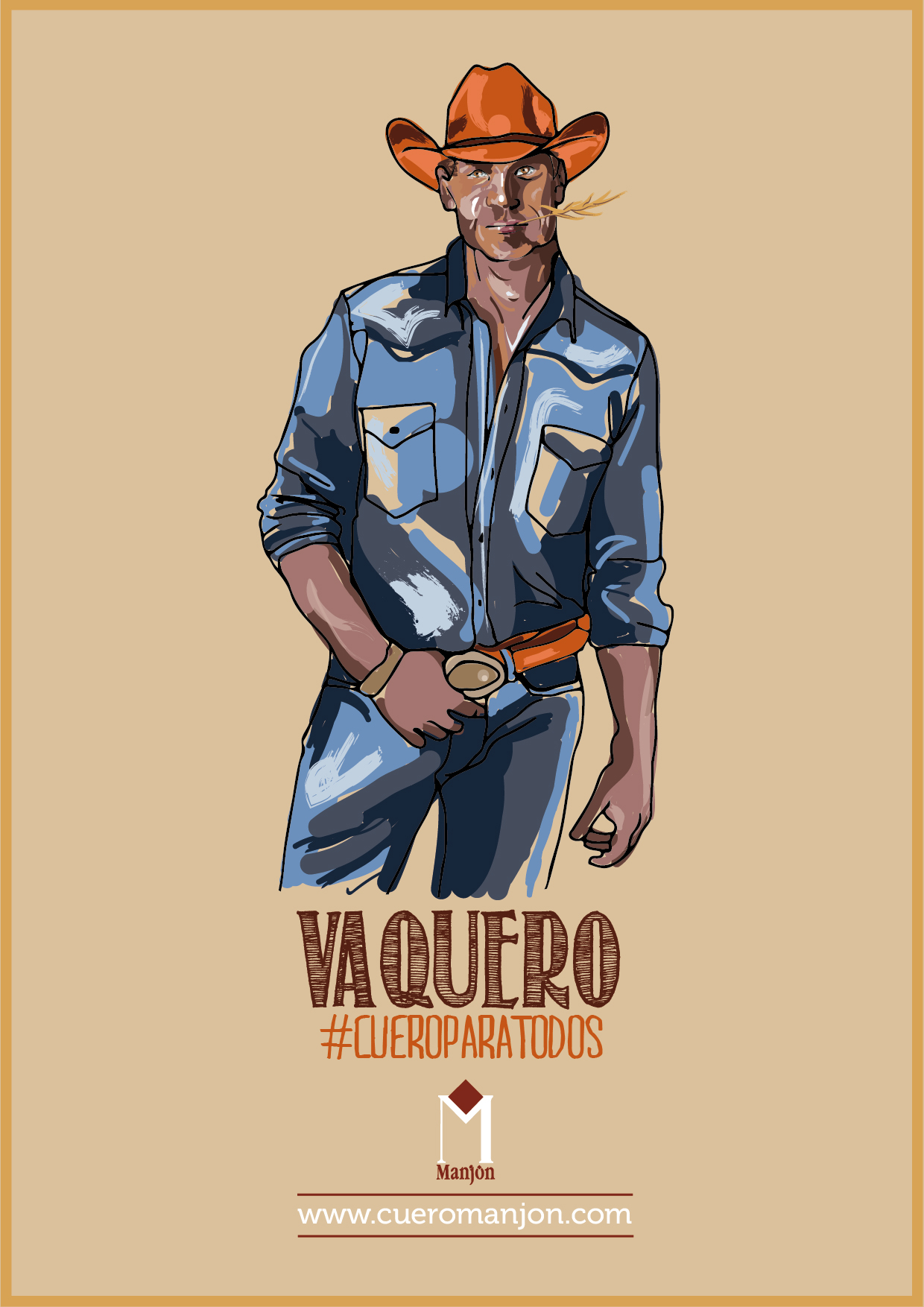The image is a stylized advertisement featuring a drawing of a classical cowboy, or "vaquero," depicted in a somewhat provocative pose. The cowboy, a white male, wears a rust-colored cowboy hat, an orange-brown leather belt with a round silver buckle, a blue collared denim shirt, and blue denim jeans. He has a piece of hay or wheat in his mouth and his thumb hooked through his belt in a relaxed manner. The art style resembles watercolor, with a solid tan background and a golden thin border around it. Below the image, the word "Vaquero" is prominently displayed in brown font, followed by the hashtag "#CuerpoParaTodos." Additionally, the trademark "Manjon" is present, alongside a maroon-colored diamond shape resting on the letter 'M.' The website "www.cuervomanjon.com" is listed below this, in white letters against a maroon bar.